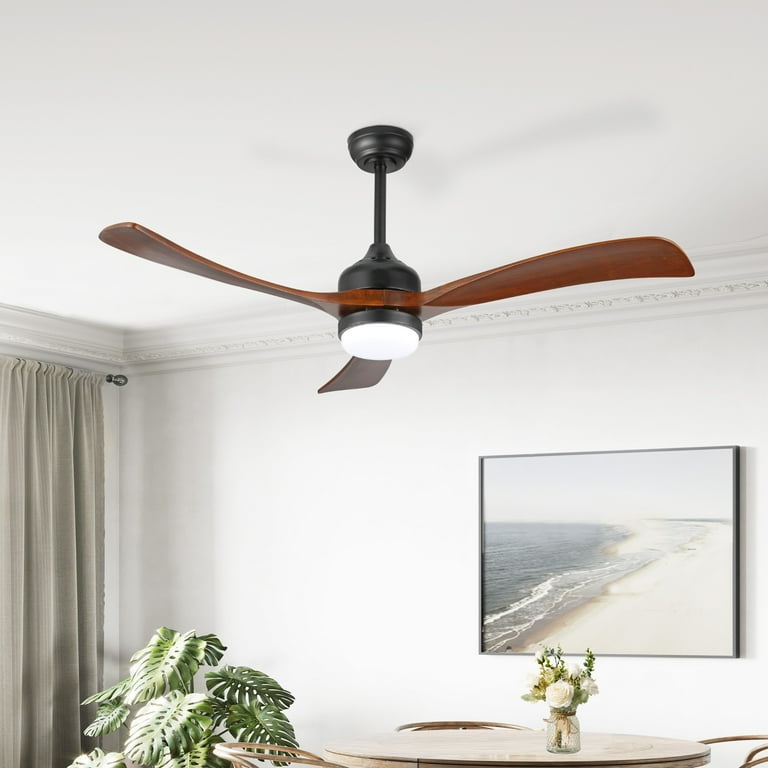The image showcases a beautifully sunlit room adorned with intricate crown molding at the ceiling. The space is dominated by a modern ceiling fan, featuring sleek, hand-carved wooden blades and black hardware, with a dome-shaped light that is illuminated. The walls are pristine white, providing a clean backdrop for a serene painting of a sunset, depicting waves crashing onto a beach shore. Just beneath this artwork are beige-gray curtains complementing the room's muted tones, partially drawn to allow the sunlight to flood in.

In the bottom left corner sits a lush Monstera plant, adding a vibrant touch of green to the setting. At the center of the room, a wooden table surrounded by several chairs offers a cozy gathering spot. Atop the table, a small pot of white roses in a clear vase filled with water enhances the room's elegance. The overall ambiance is one of modern sophistication blended with natural elements, creating a welcoming and serene interior space.